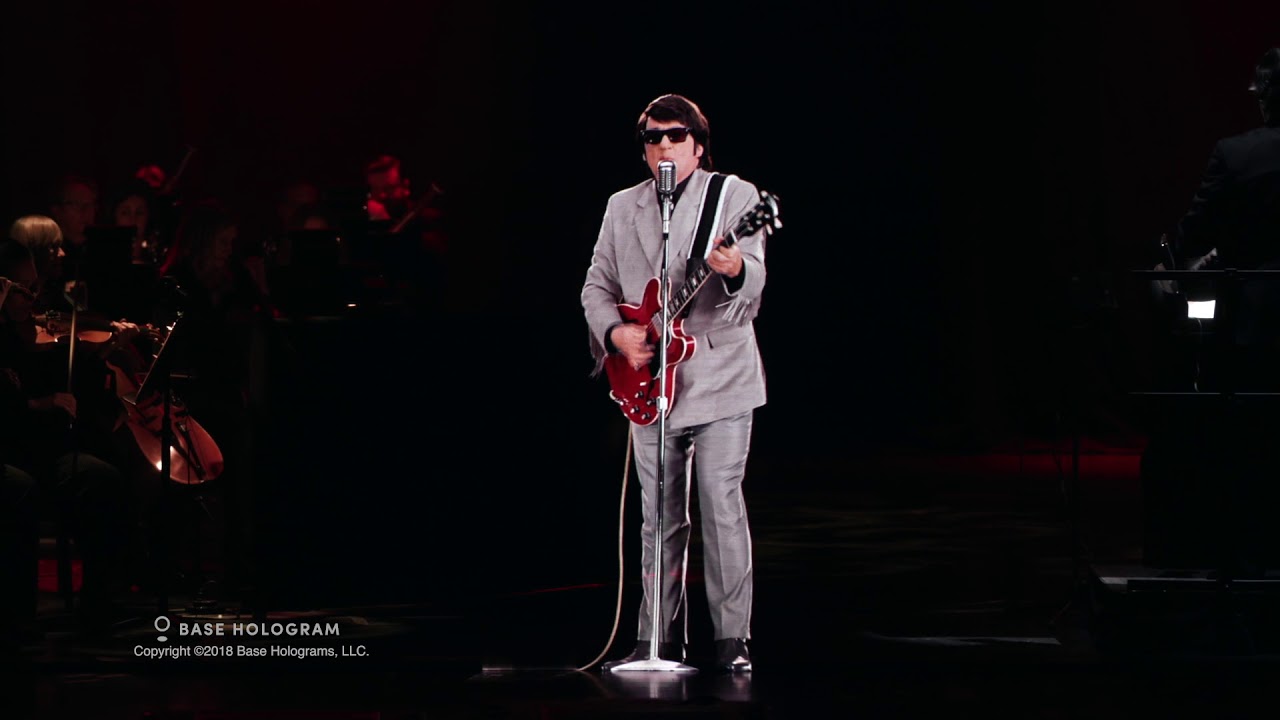This is a detailed photograph from Base Hologram 2018 depicting Roy Orbison, or more likely a hologram of him, standing center-stage. He is a white male with dark brown hair and iconic dark sunglasses, wearing a gray fitted suit over a black shirt, completed with black shoes. Orbison is captured at a slight sideways angle, playing a striking red electric guitar with a black strap, and singing into a vintage-style stand-up microphone. The stage floor and the base of the microphone stand are visible. The background is mostly blurred but reveals silhouettes of an orchestra, including a cello and possibly a violin, primarily positioned to the left-hand side of the image. To the right, there appears to be a bright, unidentifiable light, which might be related to the hologram setup. White text at the bottom left corner of the photograph reads "Base Hologram © 2018 Base Hologram LLC."